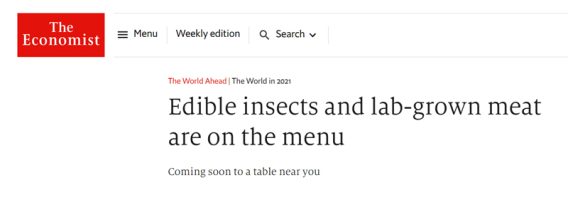This image is a screenshot from The Economist's website. At the top, there is a distinctive red rectangle with the publication's name: "The Economist," where "The" appears in smaller white text above the larger white text of "Economist." Adjacent to this, the page features a predominantly white section with three horizontal black lines representing a menu icon labeled "Menu" in black text. Next to this is the phrase "Weekly Edition," followed by a search icon in the shape of a magnifying glass.

Beneath these elements, a headline reads, "Edible insects and lab-grown meat are on the menu," with a subheading in smaller print stating, "Coming soon to a table near you." Above this headline, in red text, are the words "The World Ahead," followed by "The World in 2021." Additionally, two faint gray lines extend horizontally from the red rectangle containing "The Economist," one at the top and one at the bottom, making them barely noticeable.